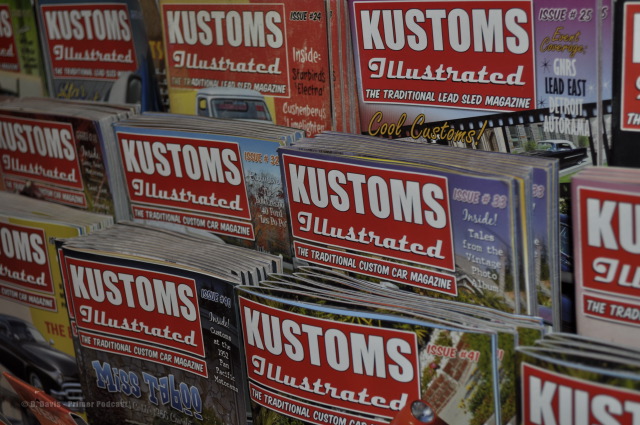The photograph depicts a magazine rack showcasing multiple issues of the same magazine titled "Kustoms Illustrated: The Traditional Lead Sled Magazine." The cover of each magazine features a red rectangle in either the upper left or upper right corner with the title "K-U-S-T-O-M-S Illustrated" in white cursive script. The magazines are arranged in three rows, each row containing different issues, with some slight variations in the cover details. The top row includes issues 24 and 25, the middle row displays issues 32 and 33, and the bottom row features issues 40 and 41. While some magazines on the far left and right are partially obscured, the central issues are clearly visible. Issue 25 highlights "G-H-R-S that leads east Detroit," and issue 32 includes a story titled "Tales from the…" although the text is partially obscured.